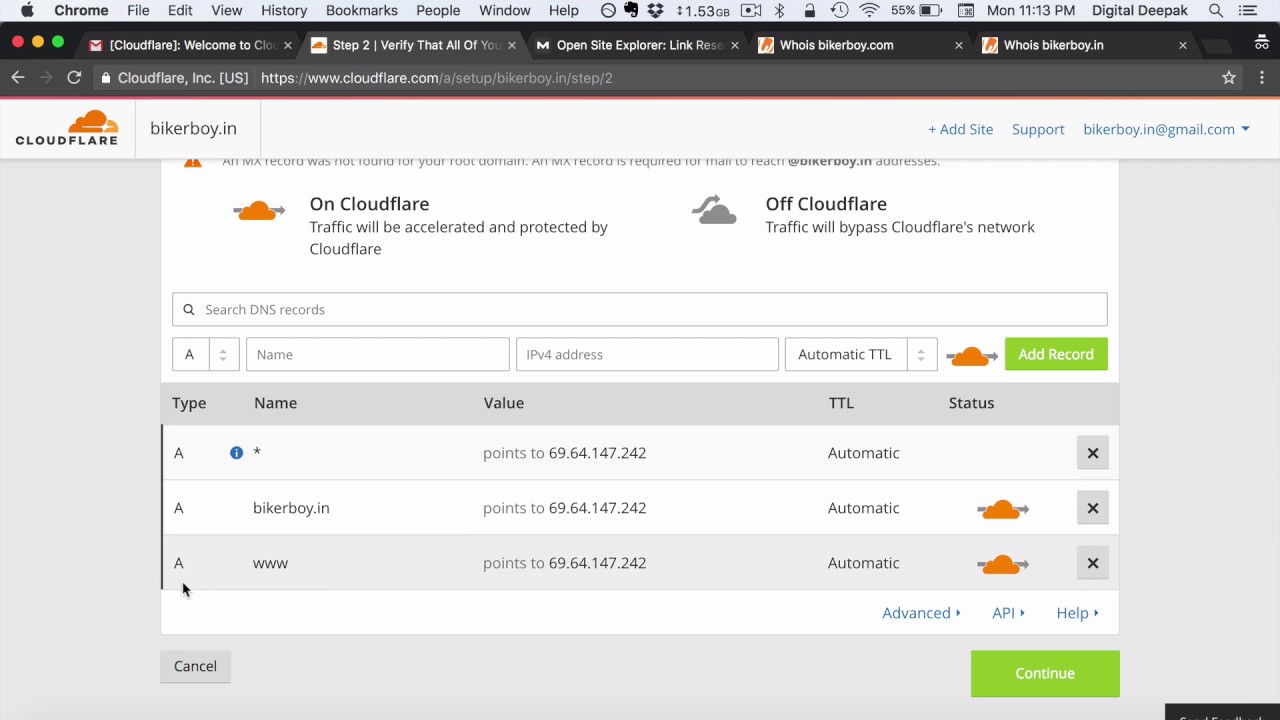The image is a screenshot of a Mac computer screen showing a Chrome web browser open to the Cloudflare website. The format is landscape, wider than it is tall. The familiar Mac icon is visible in the upper left-hand corner, along with a grey toolbar at the top displaying the text: File, Edit, View, History, Bookmarks, People, Window, and Help. The current time is indicated as 11:13 PM on a Monday.

The user, logged in as DigitalDepak, is navigating the Cloudflare Inc. (US) website, specifically on the DNS records panel. The URL shown is www.cloudflare.com. The user appears to be in the process of pointing their domain to a web service named Biker Boy. The DNS records panel reveals the details necessary for directing the domain name to the correct IP addresses, a critical step in setting up a website that links domain names to their respective web servers.